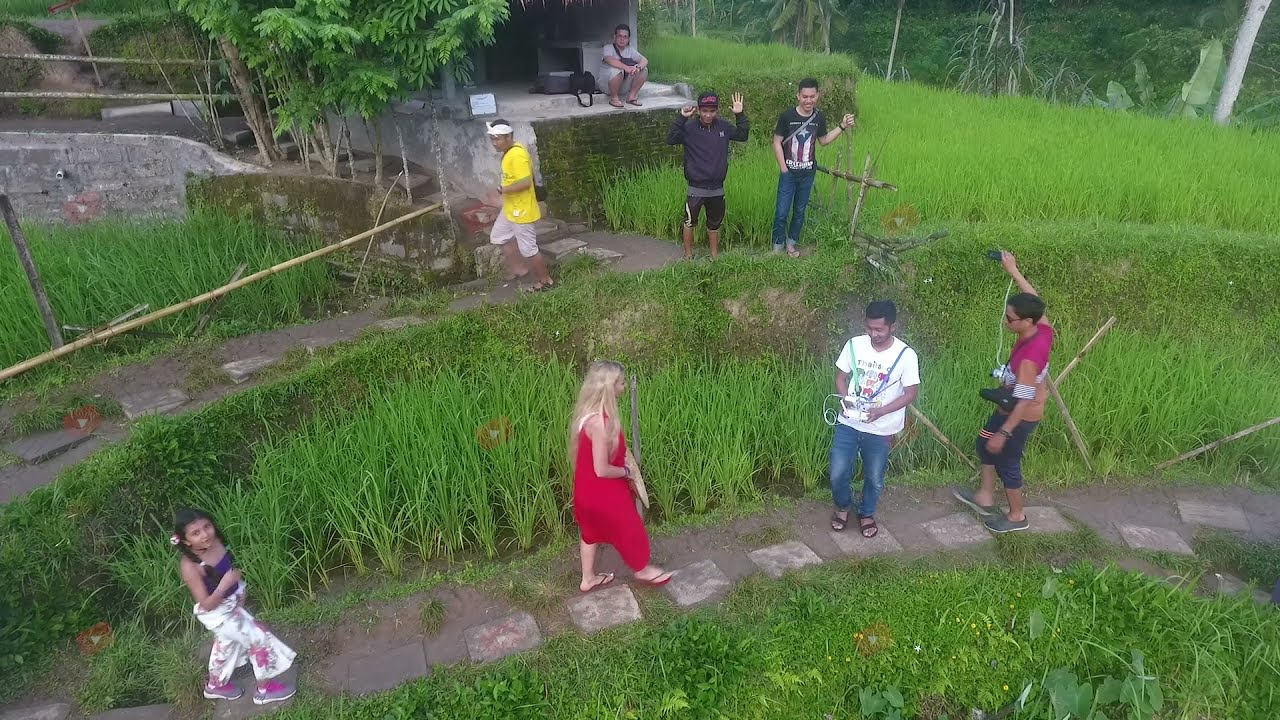The image captures an outdoor scene on a bright day featuring seven people distributed across various walking paths made of square stone pavers surrounded by tall green grass. On the lower walking path, starting from the left, there is a young girl with dark pigtails wearing a purple shirt and light-colored floral pants. Next to her is a woman in a red dress with blonde hair. To their right, a man in a white shirt and blue jeans is seen alongside another man wearing a magenta shirt with dark hair and dark glasses. Behind them, on a slightly elevated walking path, three more people are visible: a man in a yellow shirt, another man in a black jacket raising one hand, and a third man wearing a shirt displaying red, white, and blue colors. In the background, further up and slightly behind the elevated path, sits a man in a gray shirt with his forearms wrapped around his legs, perched on a stone seating area. The overall setting includes lush green grassy areas around the paths.